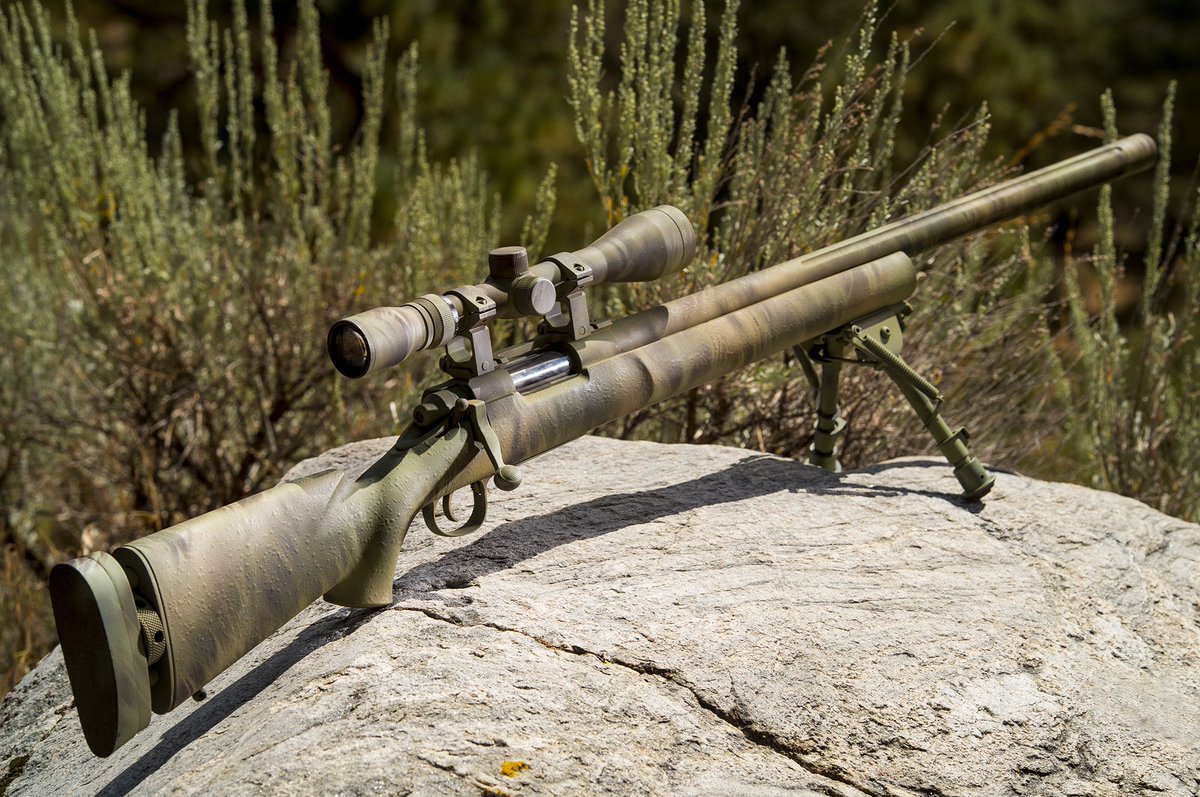The photograph captures a bolt action rifle with a long, thin, camouflaged barrel pointing towards the top right corner of the image, and its buttstock angled to the bottom left. The rifle is sturdily mounted on a green bipod attached under the barrel, which rests atop a large, light gray boulder with a prominent crack running through its center. The rifle, predominantly in a fatigue camouflage pattern of green and beige, has a standout cylinder for its bolt action that remains uncovered. The rifle features a large, advanced scope positioned above the ejection port, with a green ejection handle, and a round trigger guard. Notably, the buttstock is slightly extended, creating a visible gap between the stock and its padding. Surrounding the rock are some green weeds and brush, while the background remains slightly blurry with a greenish hue, indicating vegetation. The overall scene suggests a military context, enhanced by the imposing presence of the boulder and detailed camouflage of the rifle.